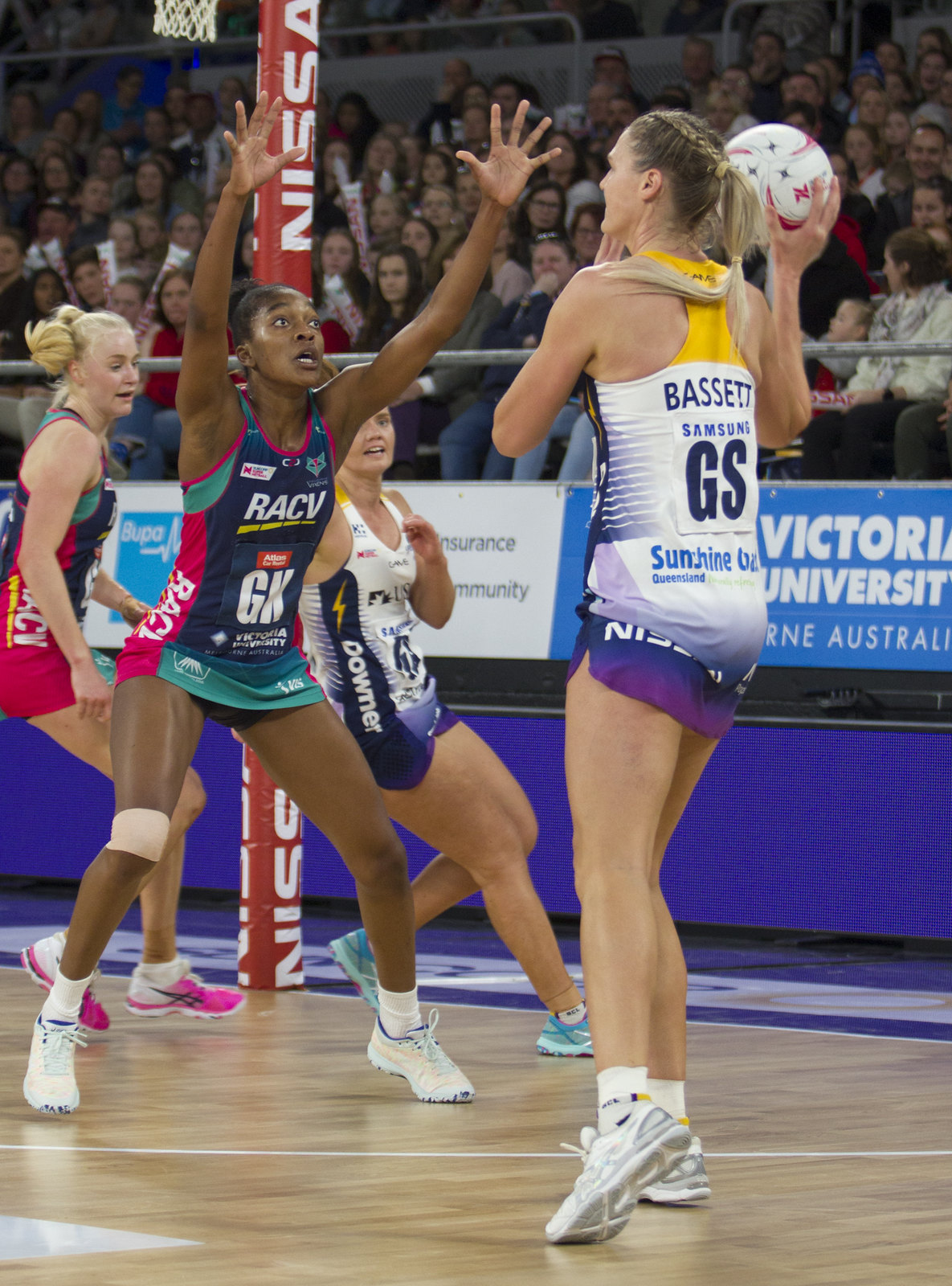The image is a tall, rectangular photo capturing an intense moment during a women's volleyball game. Four women are prominently featured on the court, which has a light brown wooden floor with white curved lines painted on it, and is situated at the bottom of the image indicating the edge of the court. In the background, beyond the floor, there is a purple barrier topped with a blue and white horizontal advertisement. Rows of spectators are visible, seated in the distant bleachers.

In the foreground on the right, there is a very tall blonde woman with white skin, facing away from the camera. She is donning a yellow, white, and purple tank top paired with shorts and is holding a white and red volleyball in her right hand. Directly in front of her is a tall black woman dressed in a striking blue, red, and green volleyball uniform. Her legs are apart, and she has both her hands raised high in the air, as if preparing to block or receive the ball. Her expression appears focused, looking directly at her teammate or opponent.

To the left and slightly behind this pair are two other female players in various action poses, suggesting that they are halting their movements, with knees bent and arms outstretched to maintain balance. The backdrop of the image includes an array of blue banners, adding to the vivid and energetic atmosphere of the game.